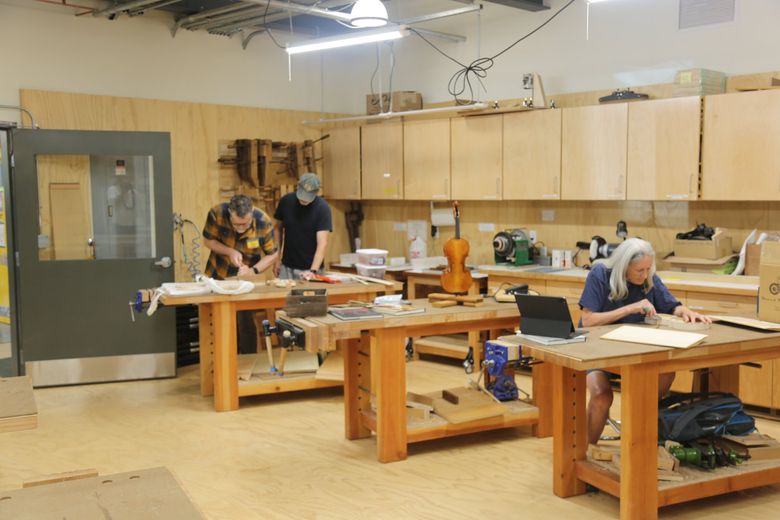In the image, a well-organized workshop with light brown wooden cabinets, paneling, and workbenches is depicted. The room features three wooden workstations lined up from the back to the front. The first workbench, situated at the back, is occupied by two men collaborating on a project. The man on the left, wearing a blue and yellow plaid shirt, holds a tool in his hands and concentrates on his work, while his younger companion in a black t-shirt and grey ball cap leans in to assist. The central workstation holds a collection of books, a wooden cello, a wooden box with unspecified contents, and several other woodworking items. The foremost workbench is dominated by an elderly woman with long white hair, dressed in a blue shirt. She sits on a stool, absorbed in measuring something with her hands. Next to her, a black tablet is propped up, suggesting she might be using it for reference. Scattered around the workshop are various tools, cups, and equipment placed on shelves and sideboards, ensuring a functional and resourceful environment for the artisans within. An open gray door with a rectangular clear window is visible on the far left, adding an element of accessibility and light to the bustling workspace.